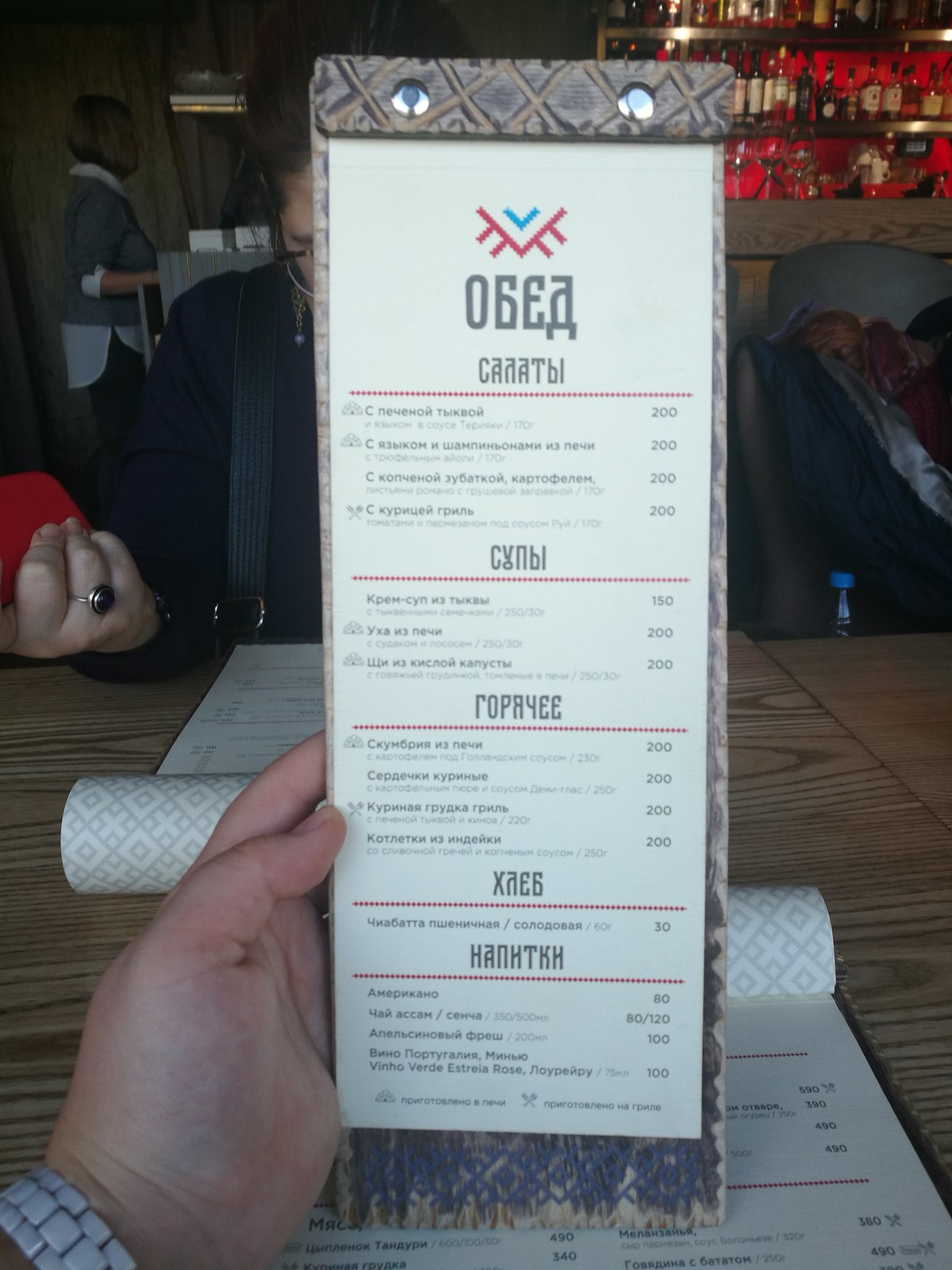In this detailed photograph taken at a restaurant, the primary focus is a tall, skinny, rectangular menu that appears to be written in Cyrillic, possibly Russian. The top of the menu features a distinct gray section adorned with a pattern of yellow X’s, secured by two silver bolts attaching it to its cover. The menu’s color scheme presents a clean white background, prominently showcasing the restaurant’s logo, which consists of an upside-down triangle with two slashes on each side and a turquoise V shape entering the triangle.

At the top of the menu is the restaurant’s name in Cyrillic, though it is not easily pronounced. The menu itself is divided into four sections, each likely listing food or beverage offerings. A man’s hand is holding the menu, revealing his white skin tone and a silver wristwatch on his left wrist. Below this slender menu, another wider menu can be seen lying flat on the table, which appears to be wooden, adding a warm, rustic touch to the setting.